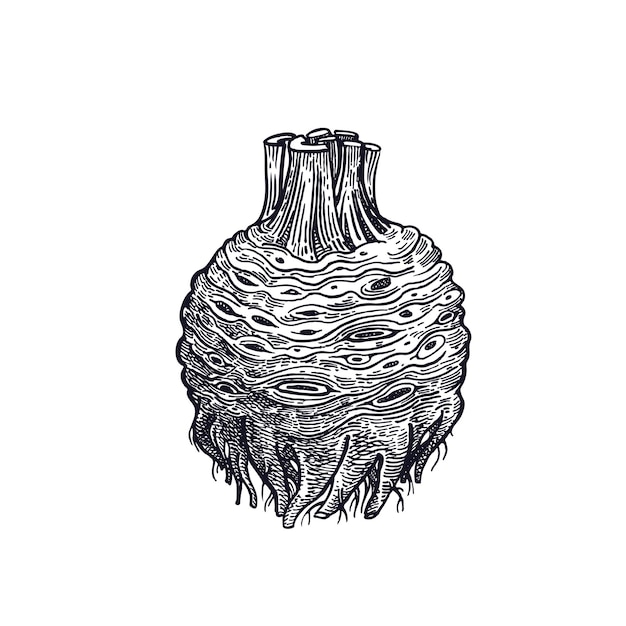This black-and-white pen and ink drawing portrays a dense, intricate root system of a root vegetable, reminiscent of a celery plant when cut close to the bottom of the stalk. The central root ball is slightly rounded, with slender, finger-like roots descending and terminating in fine, hair-like filaments. The detailed illustration includes various intricacies such as curves, openings, and orifices, giving it a somewhat grotesque, almost horror-like appearance. This root ball appears to be wrapped around in a circular manner, with the top trimmed or cut, similar to a harvested vegetable with woody stubs. The illustration, reminiscent of a woodcut or ink print, showcases a stark monochromatic contrast, enhancing the eerie, eye-like shapes resembling frog or goat eyes scattered across the root ball's surface.